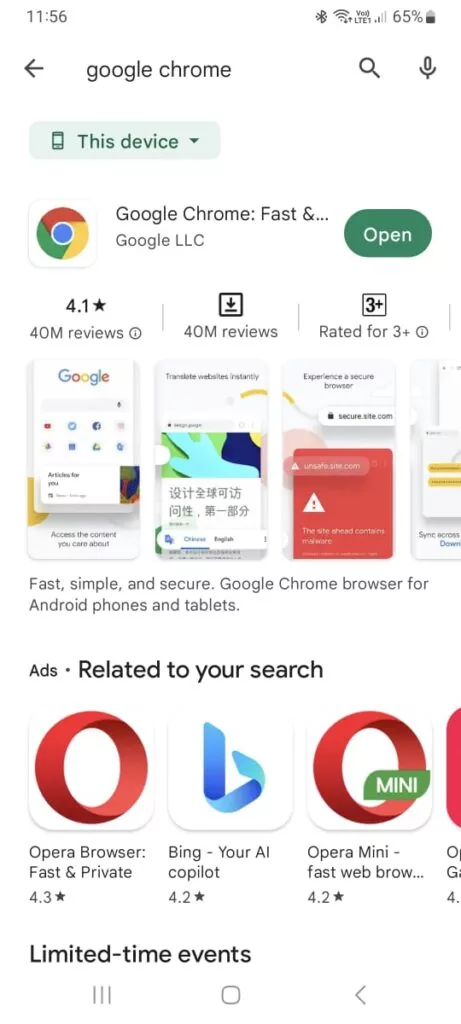Screenshot from a cell phone display. The top section shows the notification bar indicating the time as 11:56, with icons for Bluetooth, Wi-Fi, and a battery level at 65%. The main content captures a search query and results page for Google Chrome. The search result highlights Google Chrome, described as "fast and..." by Google LLC, with an "Open" button and the recognizable Chrome icon—a circle segmented in red, yellow, and green, with a blue center. Below the icon, it displays a rating of 4.1 stars from 40 million reviews and rated suitable for ages 3 and up.

Further down, various screenshots showcase Google Chrome in different languages, emphasizing its speed, simplicity, and security as a browser for Android phones and tablets. The device also lists other browsers related to the search:

1. Opera Browser - fast and private, 4.3 stars, icon featuring a red circle in a white square.
2. Bing – your AI copilot, 4.2 stars, with a white icon displaying a stylized lowercase 'b'.
3. Opera Mini – fast web browser, 4.2 stars, showing the Opera logo with a small green "Mini" banner at the top.

The image is a screenshot, with no people present.